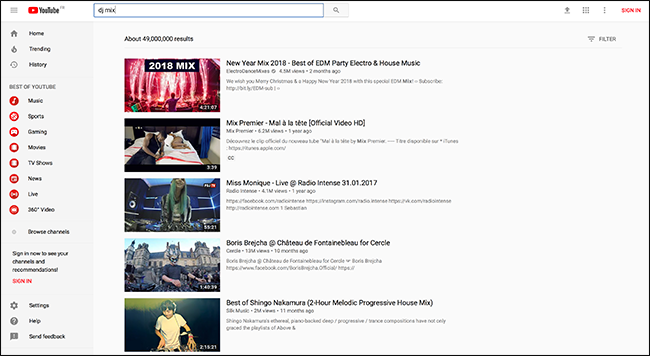This image captures the interface of the popular YouTube website. In the top left corner, the recognizable YouTube logo is prominently displayed along with the label "YouTube." Directly beneath the logo are various menu options, each accompanied by a red icon. These options include: Home, Trending, History, The Best of YouTube, Music, Sports, Gaming, Movies, TV Shows, News, Live, and 360 Videos. 

Further down, the sidebar features a “Browse Channels” section. Just below this, a prompt encourages users to sign in with the text: "Sign in now to see your channels and recommendations." A prominent red "Sign In" button follows this prompt. Additional options for Settings, Help, and Send Feedback are listed at the bottom of the sidebar.

At the top of the page, the search bar contains a query for a mix, yielding several search results. The first result is titled "New Year Mix 2018 - Best of EDM, Party, Electro & House Music," accompanied by its corresponding metadata. The second listing is labeled "Mix Premiere" with further details, though some of the text is unreadable. The following entry is "Miss Monique Live at Radio Intense 31/01/2017" including additional information below. Next in the lineup is "Boris Brejcha at Château de Fontainebleau for Cercle," also paired with its respective details. Finally, there is "Best of Shingo Nakamura 2-Hour Melodic Progressive House Mix," complete with its descriptive information below.